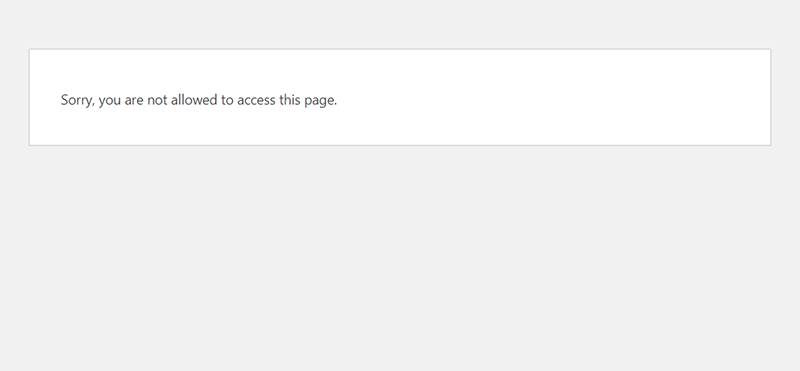A simple, landscape-oriented computer screen image is depicted, with dimensions approximately twice as wide as it is tall. The background is a light gray color. Dominating the upper third of the image is a long rectangular white box containing a message. The white box, which occupies about 25-30% of the image’s height, is bordered by narrow gray margins on both its left and right sides, each taking up between 5% and 10% of the image's width.

Inside the white box, near the left edge but not touching, is left-aligned gray text that reads: "Sorry, you are not allowed to access this page." The 'S' in "Sorry" is capitalized while the rest of the text is in lowercase. There is considerably more empty space to the right of the text within the white box. The remainder of the image, beneath the white box, consists of the same light gray background. The overall aesthetic is minimalistic and emphasizes the access restriction message.